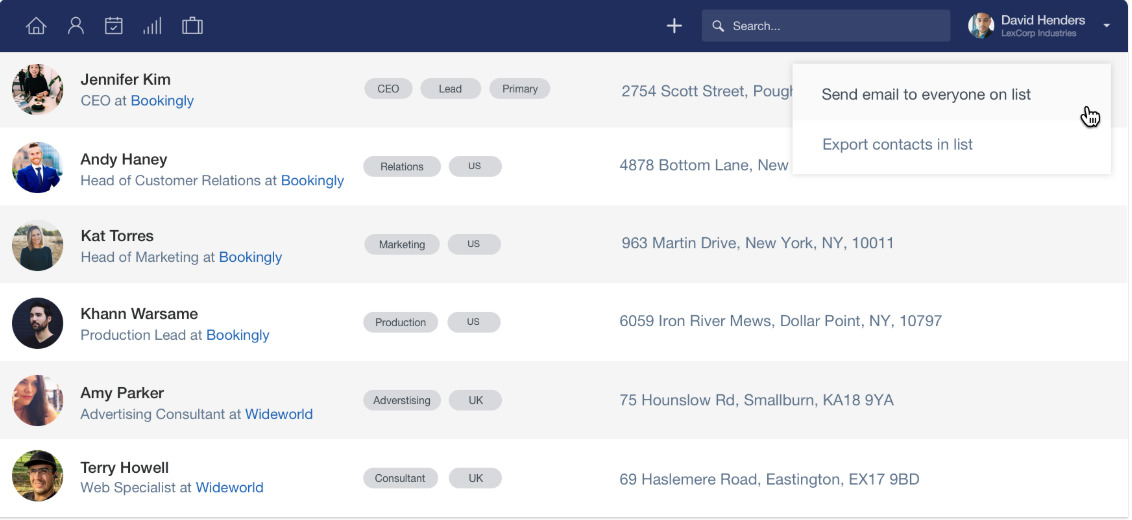This image depicts the contact section of the David Henderson LexCorp Industries website. At the top, there is a standard navigation bar with various sections of the website. The main content area focuses on contacts within the company, specifically showcasing a list of key personnel from Bookingly.

On the right-hand side of the screen, there is a small window with options to either "Send an email to everyone on the list" or "Export contacts in list."

The contact list includes detailed profiles for several individuals:
- Jennifer Kim: CEO at Bookingly. Her profile includes her email address and headshot.
- Ian Dehaney: Head of Customer Relations at Bookingly. His profile includes his email address and headshot.
- Kat Torres, Khan Warsame, Amy Parker, and Terry Howell: All are listed with their respective email addresses and headshots.

To the right of Jennifer Kim’s name, her title, "CEO," is specified, while the titles for the other individuals are not mentioned. Below the list, there are categories for various departments such as Relations, Marketing, Production, Advertising, and Consulting, implying organizational roles and divisions within the company.